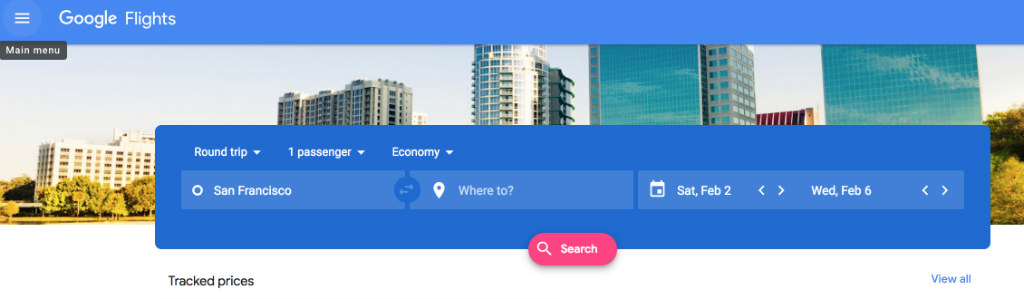The image is a screenshot of the Google Flights website. The navigation bar at the top is blue with white text displaying "Google Flights," and a hamburger menu labeled "Main Menu" appears in the far left corner with white text on a black background. The main header features a cityscape background, overlaid with the flight booking interface. There are three drop-down menus: the selected options include "Round Trip," "1 Passenger Economy," and "From San Francisco to [destination]." Travel dates from February 2nd to February 6th are displayed. These fields have a blue background with white text, and at the bottom of the interface is a red "Search" button with white text.